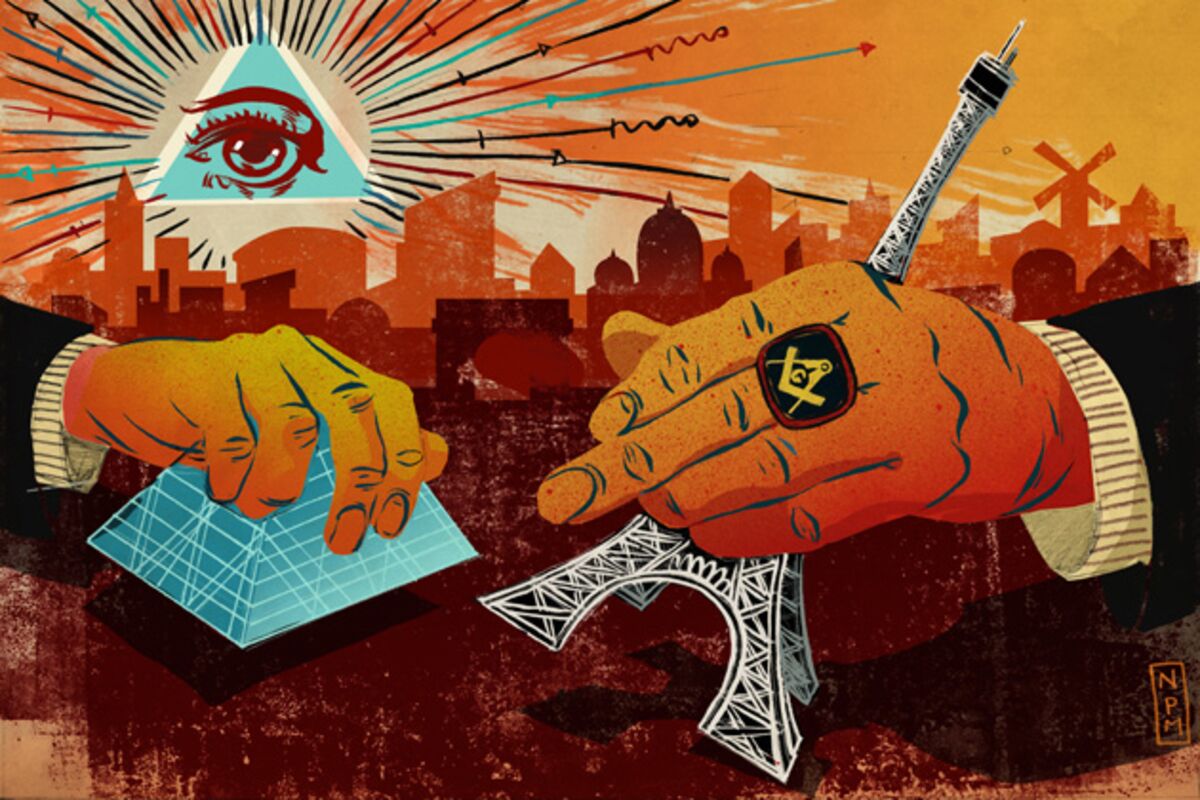This landscape-oriented painting features a striking cityscape in the background, depicted in shades of orange and fading into dark reds. Dominating the sky is an orange hue, with a prominent blue triangle outlined in white, housing a brown eye at its center. Radiating from it are multicolored rays in blue, black, and orange, adding a surreal touch to the scene. 

In the foreground, two large hands emerge, both adorned in dark suit sleeves with white shirts peeking out, suggesting they belong to the same figure. The left hand holds a blue triangular pyramidion by its top, while the right hand grasps the black-and-white Eiffel Tower at an angle. Notably, the right middle finger features a significant ring, black with a red border and a yellow Masonic crest, denoting a deeper symbolic meaning. The initials "N.P.M." are discreetly placed in the bottom right corner, hinting at the artist's identity.